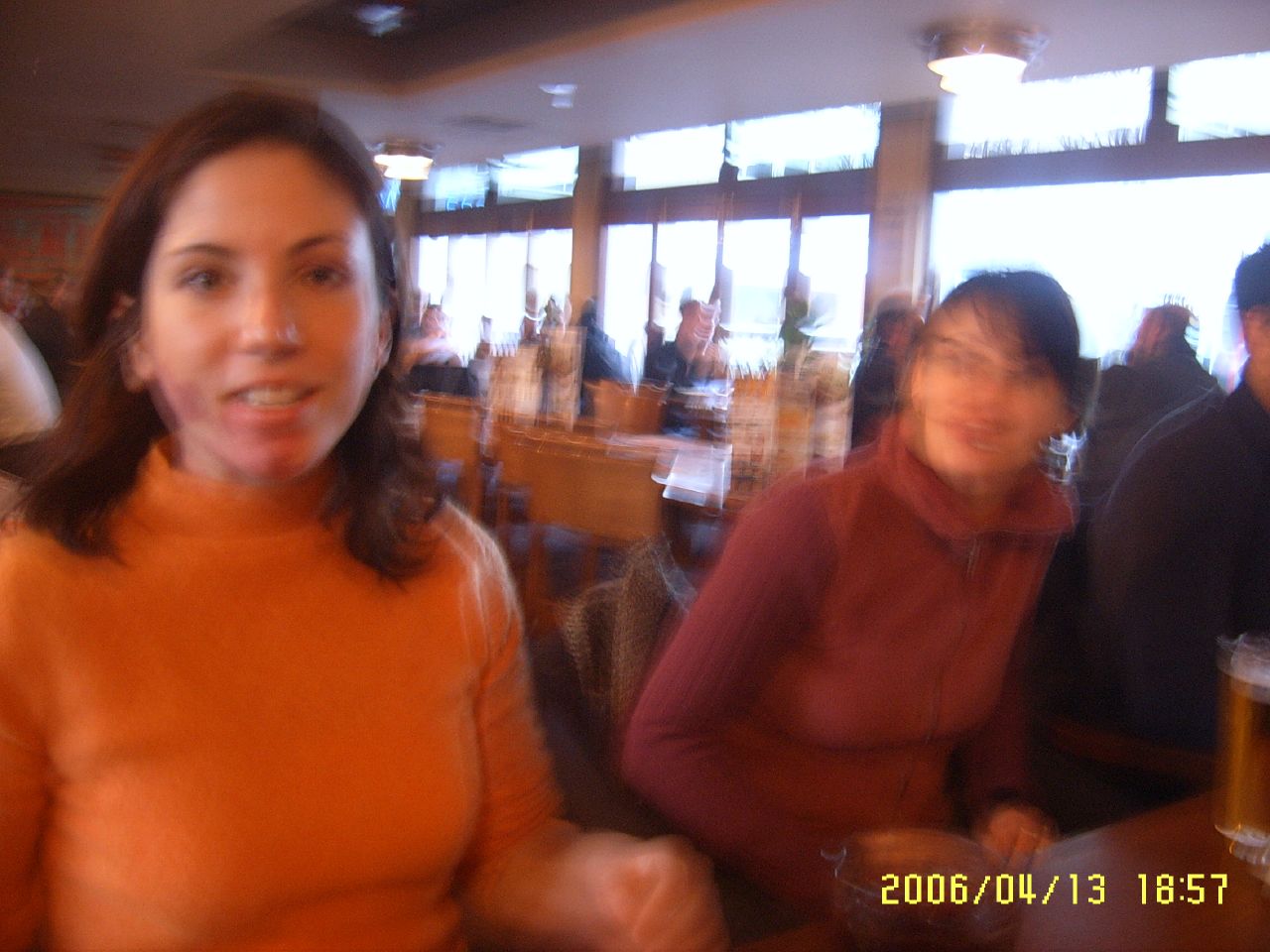This photograph, timestamped in yellow "2006/04/13 18:57" at the bottom right, appears to have been taken with an old digital or disposable camera, adding a nostalgic touch. Captured in a bar-restaurant, the image is quite blurry, likely due to an unsteady hand or possible inebriation of the photographer. The scene is set with two women seated at the bar, with wooden tables and menus visible in the background, and large windows lining the right wall of the establishment.

The woman on the left, wearing an orange turtleneck, is smiling and is slightly more in focus compared to her companion. The girl on the right dons a mauve long-sleeve shirt paired with a lighter mauve vest, but her features are indistinct due to the motion blur. Notably, her dark hair appears to be pulled back, with only her bangs in view. In front of both women, there are pints of beer, hinting at a casual, enjoyable evening. The overall scene captures a candid and lively moment between friends in a warm, convivial setting.